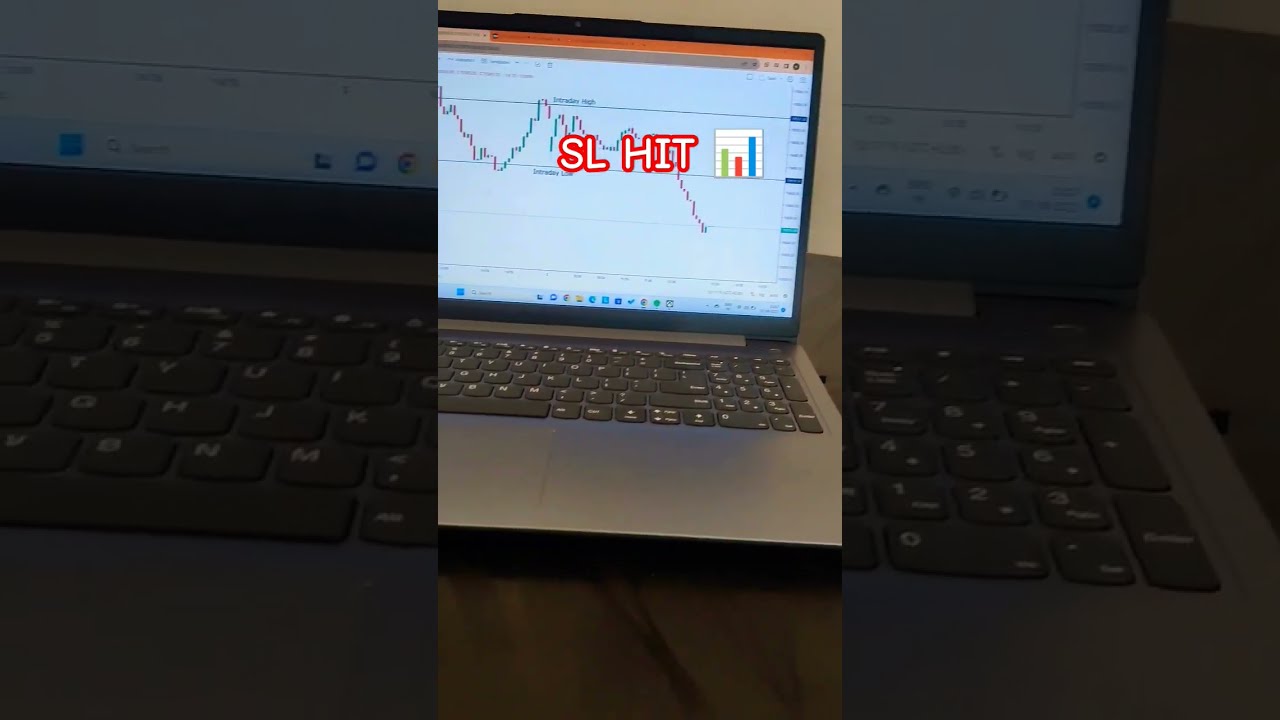The image depicts a laptop computer, open and placed on a brown table. The laptop is gray with black keys, and its screen prominently displays a bar chart with green and red vertical bars representing stock prices, which appear to follow a downward trend. The chart's background is blue, and the fluctuating lines resemble a jagged, lightning-bolt pattern, indicating volatile market activity. Overlaying the image, in bold white letters with a red border, is the text "SL HIT." This caption is not part of the screen's content but is instead superimposed onto the image. Additionally, there is a wider gray border surrounding the main image, created by enlarged, grayed-out elements of the central picture, particularly highlighting the laptop's keyboard. This border gives the impression of an inset view, emphasizing the laptop and its screen.